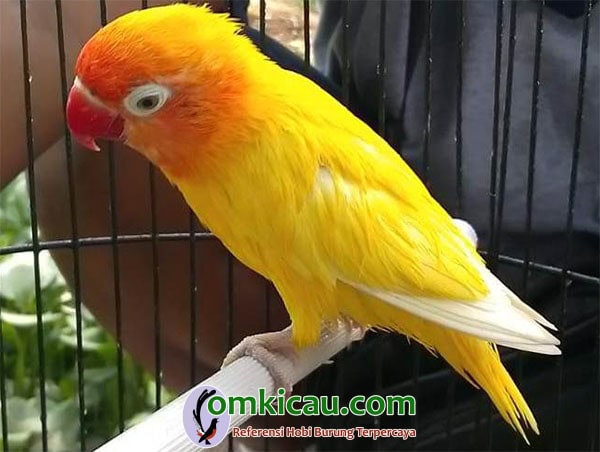The image features a detailed photograph of a vibrant parakeet perched on a textured white post inside a bird cage. The parakeet displays striking yellow feathers covering its body, with additional white feathers on its tail that stick straight out and some yellow feathers cascading slightly to the right. The bird's face is adorned with orange and red feathers, highlighted by a bright red beak and a pronounced white ring around its large eye. There is also a white ring slightly above the beak. The parakeet's feet are a grayish-beige color, gripping the post securely. The bird cage is visible behind the parakeet, notably showing bars at the back, which suggests that the cage door might be open as no bars are seen in the front. At the bottom of the image is a text overlay, featuring a website advertisement for "omkikau.com" in green letters. Beneath this, in red text, is a phrase written in a foreign language: "Referenzi Hobi Barang Terperen Kaya." In addition, a small oval logo under the letter "O" in "omkikau.com" contains an image of a bird with an upward-curving tail.